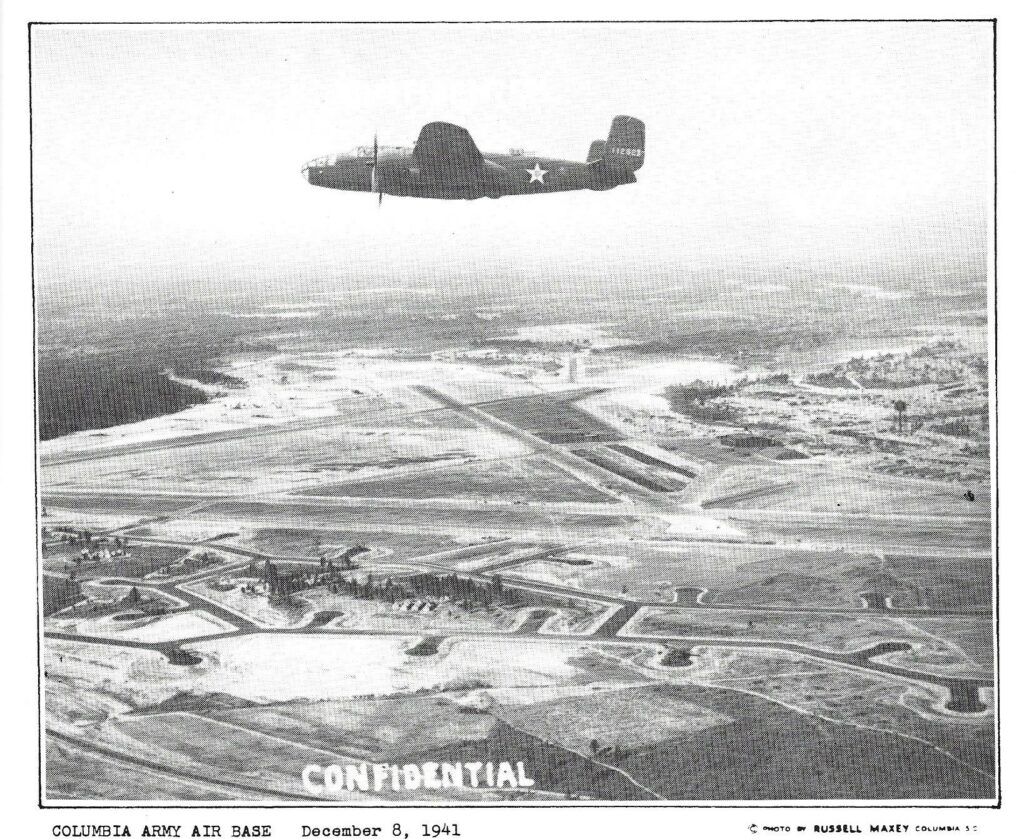This vintage black and white photograph from the World War II era captures a U.S. bomber plane in mid-flight, identifiable by the prominent white star emblem on its side. The plane is seen from a side view, highlighting its distinctive glass dome at the front, likely for a machine gunner, and a rear-facing machine gun turret. The scene reveals the aircraft flying high above Columbia Army Air Base, as indicated by the typewritten text at the bottom left of the image, which reads "Columbia Army Air Base, December 8, 1941." Adjacent to this, the bottom right credits the photograph to Russell Maxey from Columbia, SC, and stamps it with the classification "CONFIDENTIAL." The sky behind the aircraft is a stark white, providing a clear contrast to the dark-colored bomber. Below, the land appears desolate due to the grainy quality of the photo, but closer inspection reveals rural landscapes, including a runway, streets, and forested areas, giving the image a somber yet historical significance.